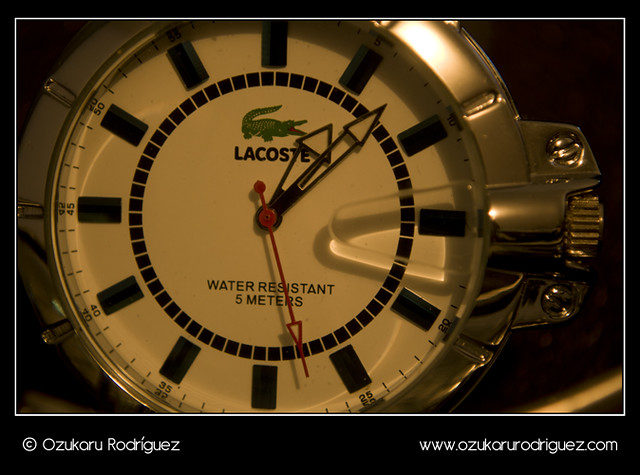The image is an advertisement featuring a detailed close-up of a Lacoste watch. The overall background is black, with a white rectangular outline situated in the upper center part. The exterior of the watch is made of a stainless steel metallic substance, with the winding stem on the right side. The watch face is white, featuring black rectangles marking each hour and smaller black squares forming a circular pattern along the inner edge. At the center is the iconic green Lacoste alligator logo with its mouth open and tail above its head, facing to the right. Below the alligator, "Lacoste" is written in black text. The watch hands are outlined in black metal with sheer sections, and the second hand is red and ends in an arrow. The image highlights the watch's water resistance up to 5 meters at the bottom. Surrounding the watch is a thicker black border at the bottom, containing the text "© Ozukaru Rodriguez" on the lower left and "www.ozukarurodriguez.com" on the lower right.